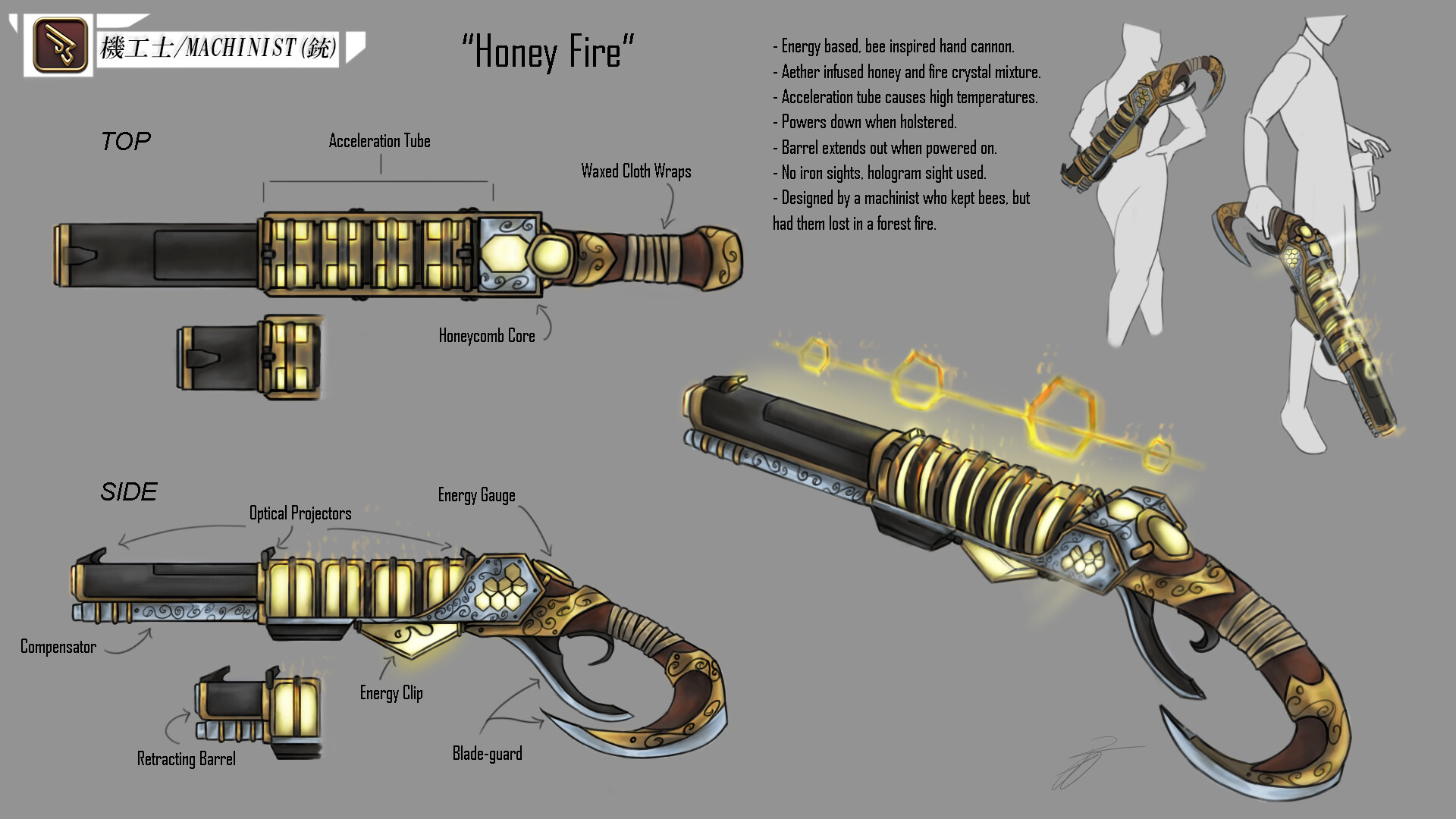The image illustrates a detailed and unique concept design of a gun titled "Honey Fire," envisioned as a fantasy weapon. The backdrop is gray. In the top left corner, a white banner bears the word "Mechanist" in black letters, with the gun's name, "Honey Fire," quoted beside it. Below this header, an overhead view of the gun is labeled with features like "acceleration tube" and "wax cloth wraps." The gun's handle, colored brown and gold, appears curved with a blade-like tip, and a small piece resembling a blade extends beneath the trigger. 

A side view of the gun in the bottom left corner confirms these details, highlighting additional components such as a compensator, optical projectors, energy gauge, energy clip, blade guard, and retracting barrel. To the right, the gun is showcased from different angles: an outline of a person carrying the gun on their back and another holding it at a slight angle. The top right corner explains the weapon's operation: it's an energy-based, bee-inspired hand cannon powered by an ether-infused honey and fire crystal mixture, featuring an acceleration tube that causes high temperatures, a hologram sight instead of iron sights, and a barrel that extends when powered on but powers down when holstered. The design is attributed to a machinist who lost their bees in a forest fire, with thematic elements like hexagonal hive shapes and glowing yellow parts on the cylinder evoking a beehive motif. At the bottom, the gun is depicted firing, with smoke circles above its barrel, emphasizing its unique features.